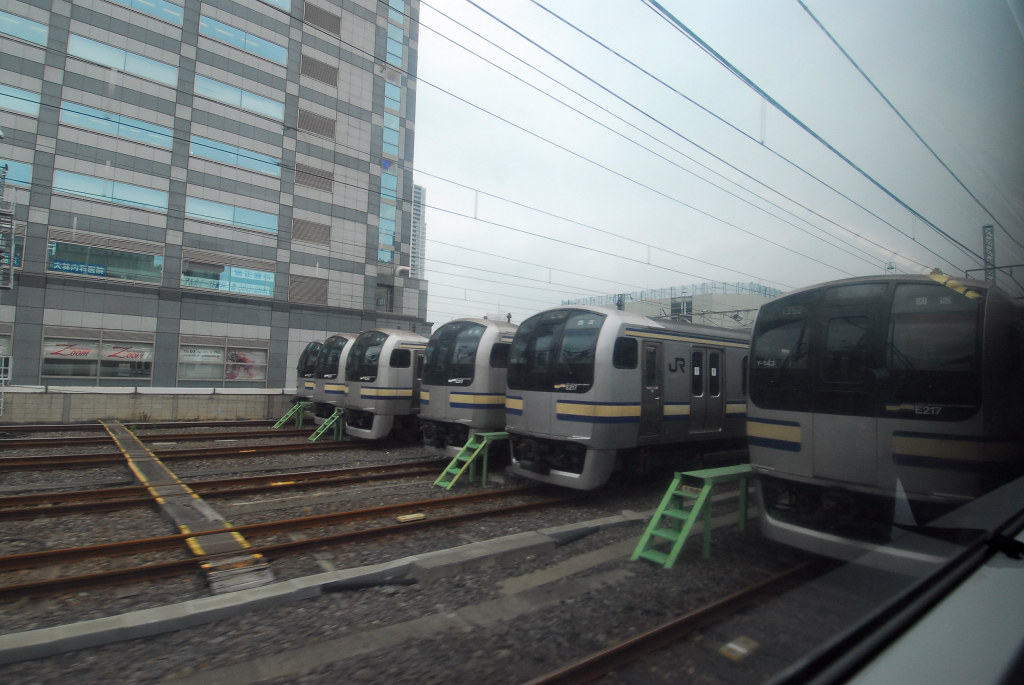The color photograph depicts a bustling train depot featuring six sleek passenger trains, all lined up meticulously, facing away towards the bottom left corner. These silver trains, possibly resembling bullet trains or airport shuttles, showcase smooth, aerodynamic designs with rectangular fronts and large black tinted windows. Identifiable by black and yellow stripes, each train is stationed on tracks paralleled by small green stairways that lead up to the platforms beside them. Overhead, a network of black electrical wires runs above each train, a crucial infrastructure for their operation. Dominating the left-hand side of the image is a significant building, around four to five stories tall, which occupies roughly a third of the image and gives context to the outdoor setting. In the immediate foreground, a wooden walkway marked with yellow lines adds yet another layer to this well-organized and dynamic scene, framed by the backdrop of a clear blue sky and the silhouette of a skyscraper.